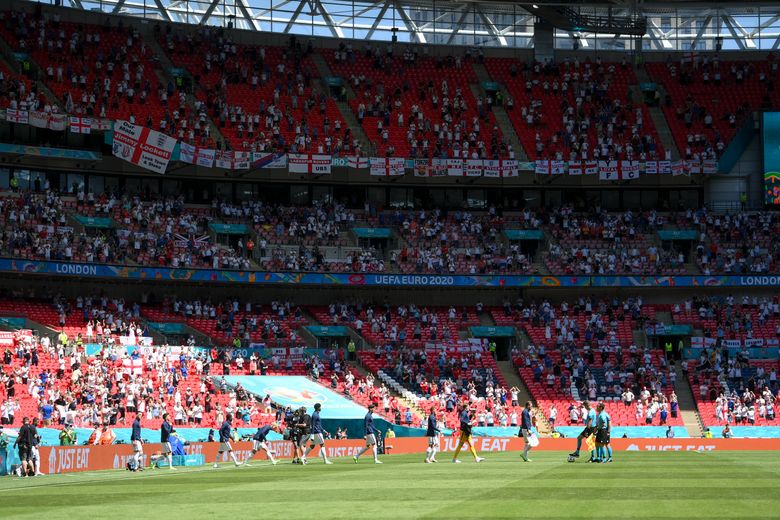This photograph captures a vibrant scene at a soccer stadium during what appears to be either the pre-game warm-up or the post-game cool down. The lush green field, with a notable lighter green patch in the bottom left, is populated with players in action, some with their feet on soccer balls. The athletes are distinguishable by their uniforms, with light blue jerseys on the right side and dark blue jerseys on the left. The players seem to be converging in the middle of the field, suggesting a significant moment of transition.

The backdrop features a grandstand with three distinct tiers of seating. The bottom section is closest to the pitch, followed by a middle section, and finally a top tier that extends towards the roof of the stadium. The seats, primarily red with hints of pink and baby blue, are only about half occupied, indicating either the anticipation of more spectators or the waning moments of the event. Despite the sparsely filled seats, the stadium buzzes with the presence of scattered fans.

Overall, the bright, sunny day enhances the crisp, vivid colors and the lively atmosphere of the scene, contributing to the energetic ambiance of this sporting event.